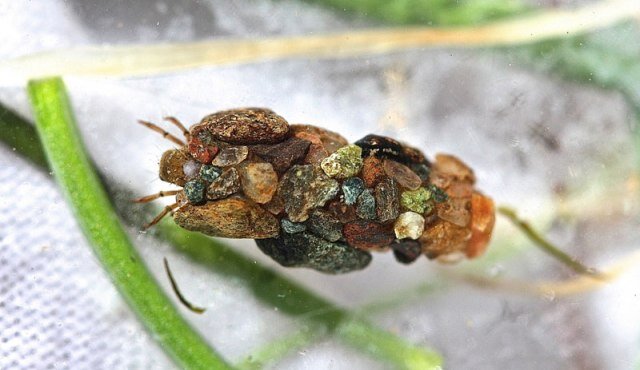The photograph is a highly detailed close-up, focusing on what seems to be an intricately camouflaged insect situated on a loosely woven white fabric. This insect is masterfully disguised to look like a small collection of diverse rocks and crystals including green, white, orange, metallic black, blue, light brown, reddish, and jade hues. The bug's body is a fascinating mosaic of these various elements, making it resemble a pile of gravel at first glance. Emerging from this assemblage, there appear to be two long green stems intertwined in the foreground, which further blends the insect into its environment. In addition, there seem to be four distinct legs protruding from beneath the "rocks" – two on each side – that resemble spider legs, while two additional long, green appendages extend behind it. The background features an out-of-focus mix of green foliage and white cloth, enhancing the illusion and depth of this remarkable camouflage.